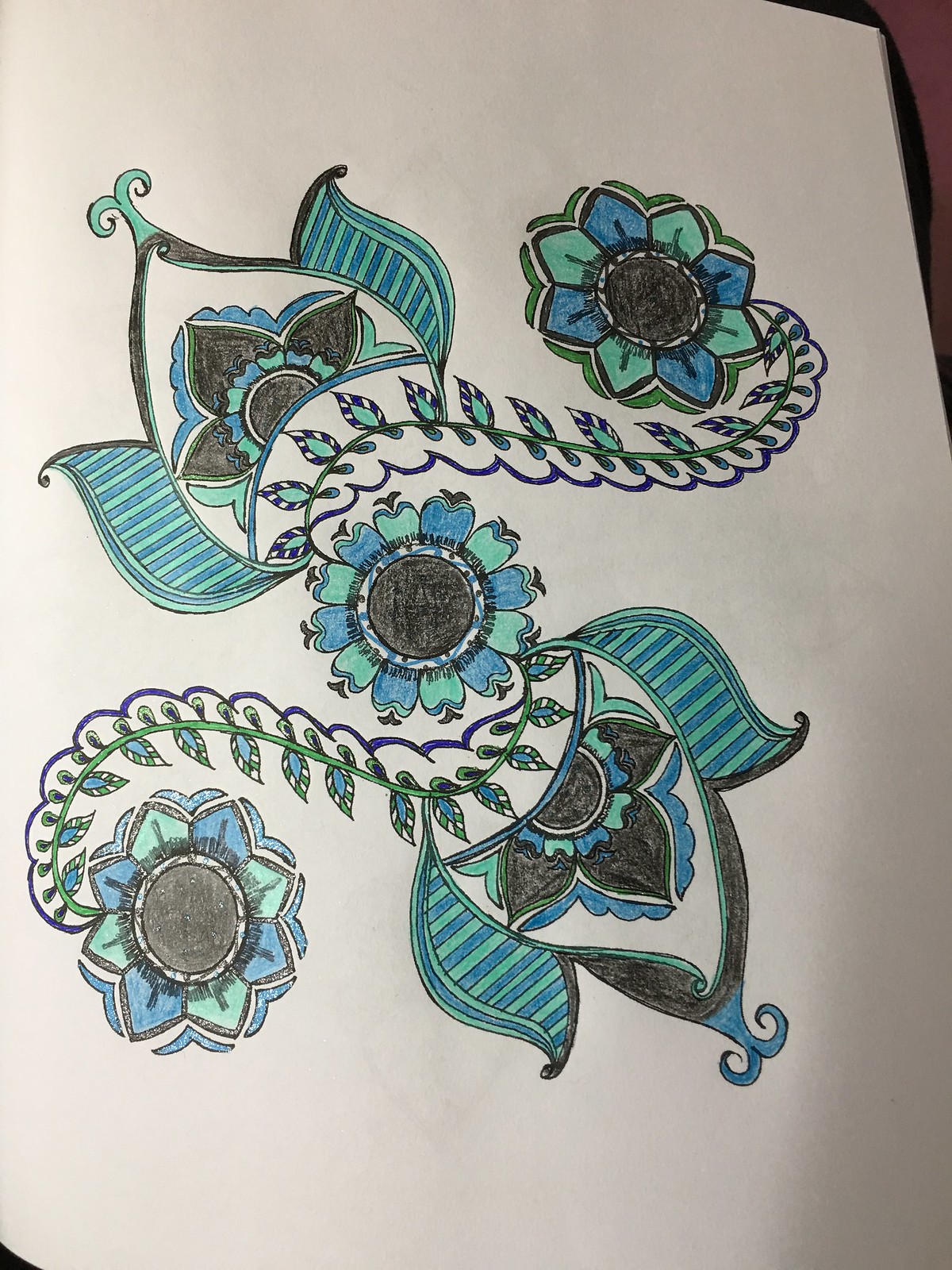This intricate colored pencil drawing on paper showcases a vibrant blue and green floral pattern with exquisitely ornate leaves. At the heart of the composition is a sunflower-like flower, featuring alternating blue and green petals encircling a black center. Two elegantly curled stems emerge from this central flower, each culminating in additional blossoms adorned with more pointed, alternating blue and green petals. Above and below the central flower, the artwork is embellished with ornate half-flower patterns in the same blue and green palette, highlighted with black accents, adding an extra touch of sophistication to this detailed and ornate piece.